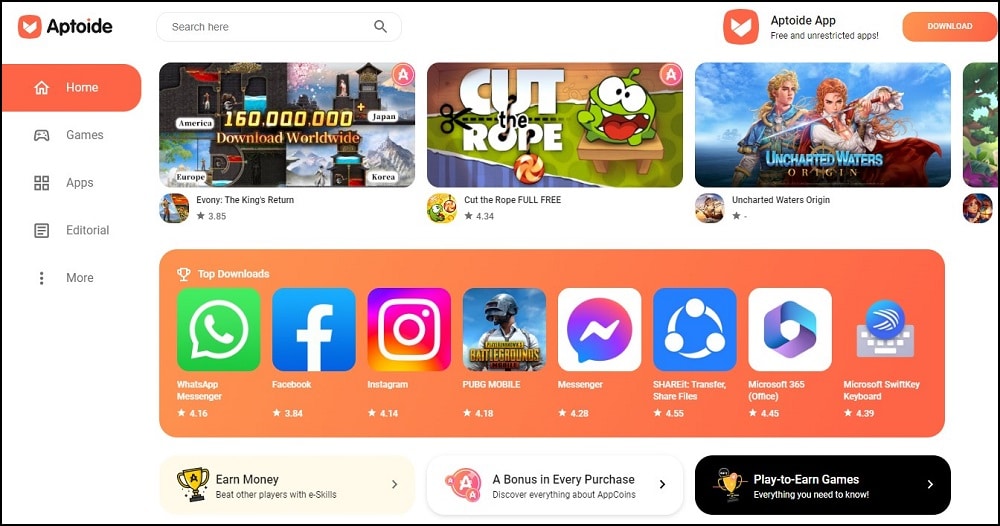The image features a white background outlined in black. In the upper left corner, there is a small red block with a white "V" and the label "Aptoide." Below this, there is a search box, followed by another red square featuring the white "V" again with the caption "Aptoide app, free and unrestricted apps." To the right, there's a red download button.

Directly underneath the Aptoide label, there's a red home button, followed by navigational options such as Games, Apps, Editorial, and a menu symbolized by three dots for more options. Along the top of the image, a banner displays various app icons and descriptions, stating "160 million downloads worldwide." Featured prominently is "Evante, The King's Return," alongside a round image. Next is "Cut the Rope," identified by its distinctive green character and noted as free. Another featured app is "Uncharted Waters: Origin," showcasing a picture of a girl and a guy on a ship. Additional partial app icons are visible below.

A prominent red box highlights "Top Downloads" with a prize icon to the left. Listed apps include WhatsApp (in green), Facebook, Instagram, Pubmobile, Messenger, Sharer, Microsoft 365, and Microsoft Surfing Keyboard.

At the bottom, there is a trophy icon with the message "Earn money, best other players with A skills," accompanied by a right arrow. Adjacent to it is a circular red badge emphasizing a bonus with every purchase, also followed by a right arrow. Lastly, a black box at the bottom reads "Play to Earn Games, Everything You Need to Know," finished with another right arrow.